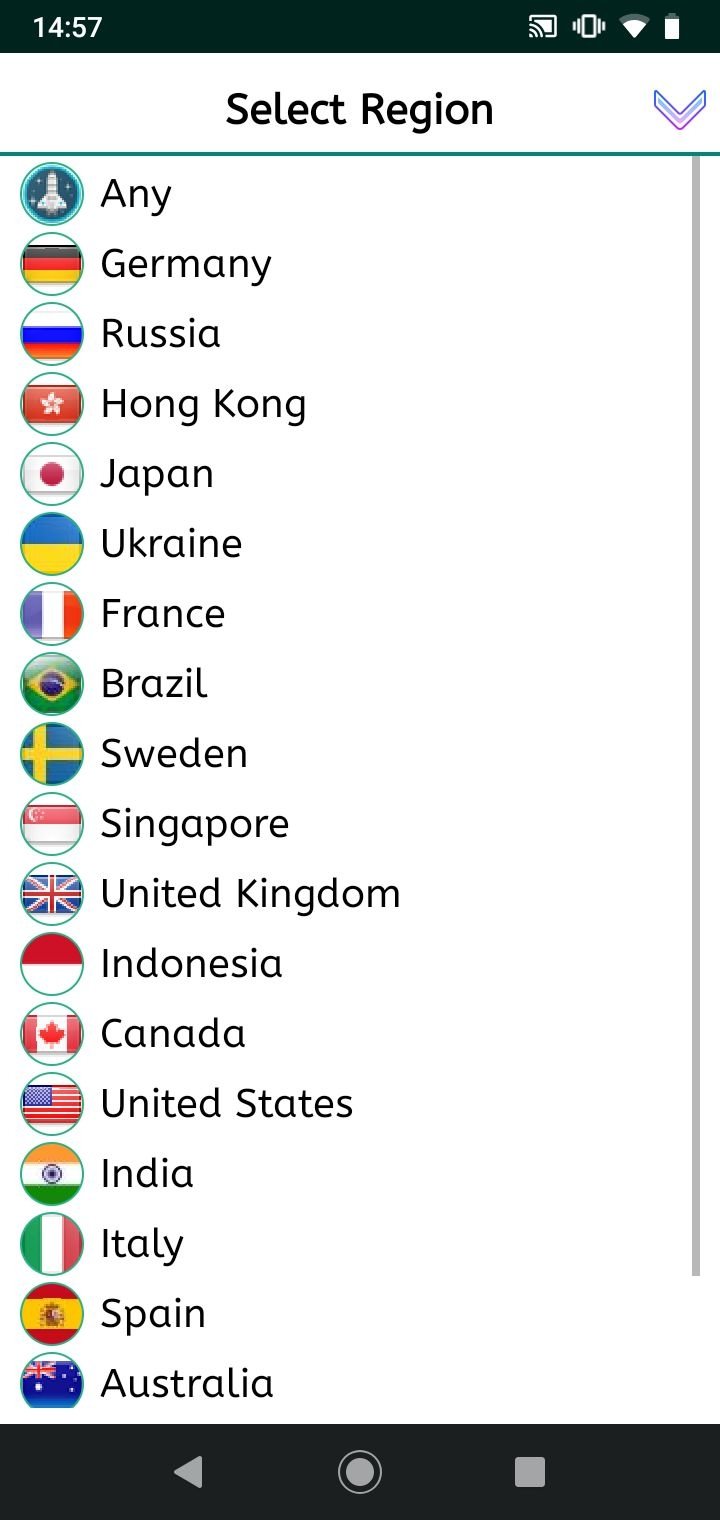This screenshot captures a region selection interface on a smartphone. At the very top of the screen, the time displayed is 14:57 (2:57 PM), and the battery level appears to be approximately 88%. The header of the page reads "Select Region," accompanied by a down arrow on the top right corner indicating a dropdown menu. The region selection menu presents a list of countries, suggesting options for configuring language or regional settings for a user profile. The visible countries are Germany, Russia, Hong Kong, Japan, Ukraine, France, Brazil, Sweden, Singapore, United Kingdom, Indonesia, Canada, United States, India, Italy, Spain, and Australia. A scrollbar on the right side implies that additional countries are listed below the visible options. At the very bottom of the screen, the smartphone's navigation bar is visible, featuring the back, home, and app switcher buttons, which are standard on most devices.